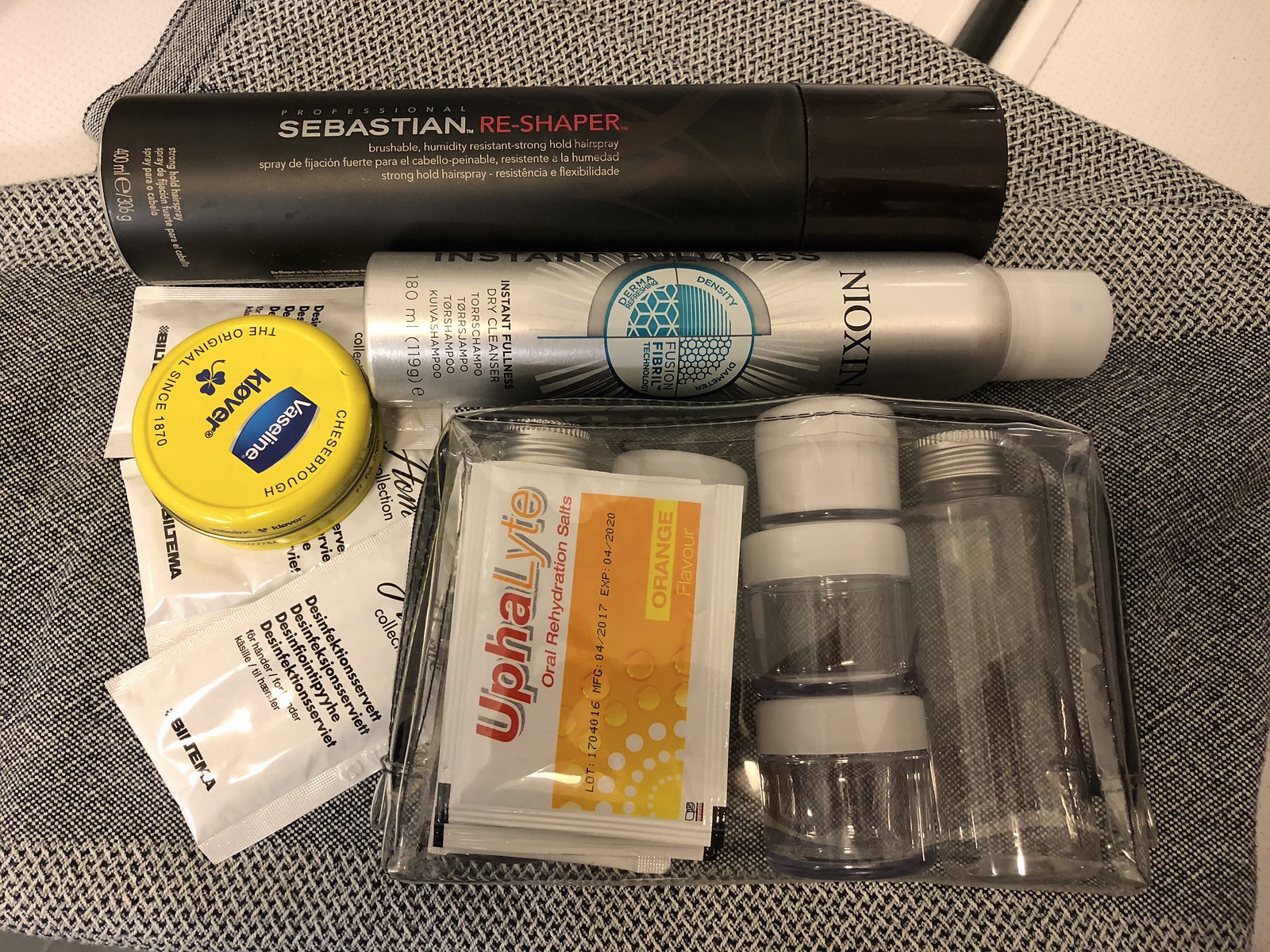On a gray mat set atop a white surface, a meticulously arranged assortment of personal care items is displayed. Central to the composition are two gray canisters of shampoo, each sleek and modern. Resting atop one of the shampoo canisters is a black canister of hairspray, adding a touch of contrast. Below the shampoo canisters lies a compact travel bag, slightly opened to reveal a sachet of oral rehydration salts peeking out. To the right of this arrangement, there is a small, narrow jar of Vaseline, notable for its compact size. Directly beneath the Vaseline are several sachets of disinfectant wipes, neatly stacked and ready for use. The overall arrangement is organized, emphasizing the essentials for personal hygiene and care.